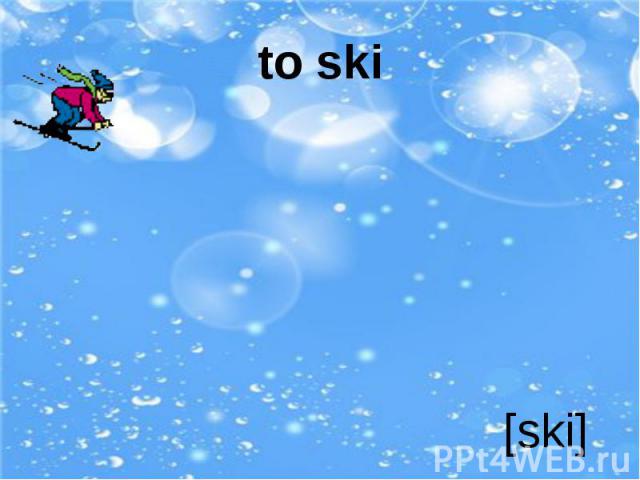The image features a dynamic and vibrant computer-generated graphic. The background is a light blue color adorned with white circles and dots that resemble water bubbles or spray, giving a lively effect. In the upper right corner, there's a lens flare, resembling a sunburst. Dominating the scene in the upper left corner is a small cartoonish skier wearing a blue hat, magenta sweater, lime green scarf fluttering behind, blue pants, and black ski boots and skis. The skier is captured in mid-action, skiing downhill. Centrally, at the top in black lowercase text, it reads "to ski". At the bottom right corner, also in lowercase, black text within brackets, it says "ski". Directly below this, in white text, appears the watermark "ppt4web.ru". This detailed illustration blends playful skiing imagery with a digitally stylized background, creating an energetic visual appeal.